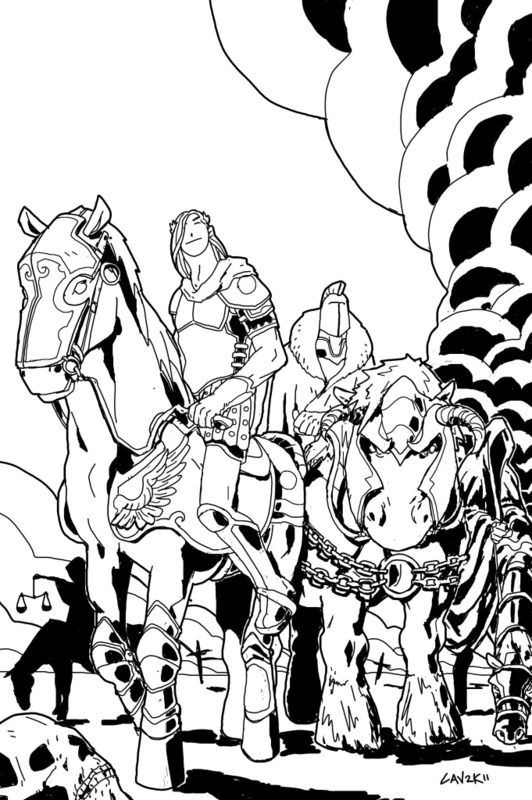The image is a vertically aligned rectangular black-and-white pen and ink drawing, styled like a comic strip or a coloring book page. Central to the composition is a knight on a horse, which is armored with metal braces on its knees and a metal covering on its face. The knight, depicted with long, straight hair, is clad in armor and appears to be holding a rope or reins in his left hand. In the foreground near the horse's hooves, lies a skull.

Directly behind this central figure is a larger and bulkier creature, potentially a rhino or a heavily armored horse, distinguished by its prominent horns and chains around its front. The rider on this creature wears a helmet, obscuring their face. Additionally, another cloaked horse with an unidentifiable rider is visible in the background.

There is an element of smoke or curving black lines in the upper right-hand corner, adding to the scene's medieval ambiance. A mysterious image of a person holding scales of justice is faintly visible in the background smoke. At the bottom of the drawing is a small, cryptic signature that reads "Tab to play 11."